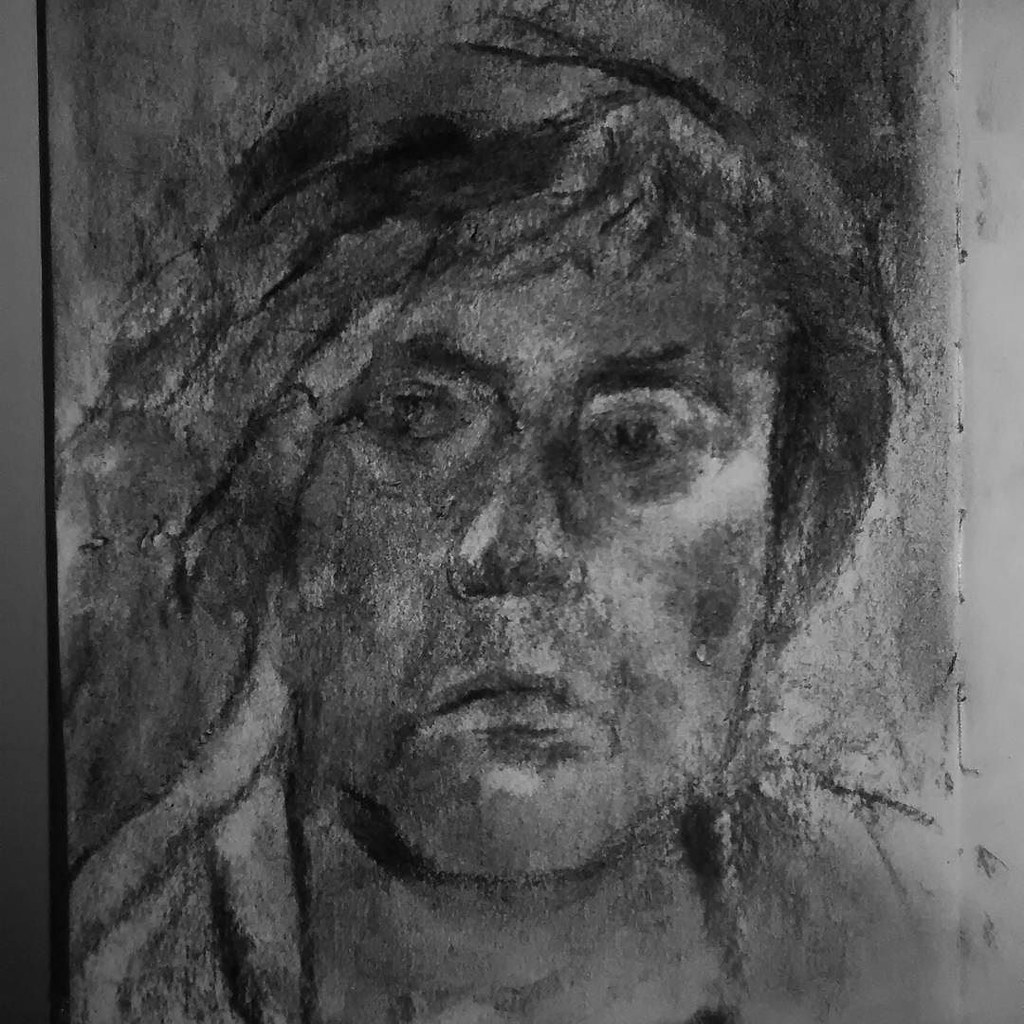A haunting image depicts a ghostly, shaded figure emerging from a blurred background. The spectral visage appears to be rendered in dark, smudged marks, possibly created using charcoal or ash, lending a somber and eerie quality. The face is marked by deep indentations suggesting sunken eyebrows and a prominent nose, with a distressed, frowning expression. Beads of sweat seem to trickle down the face, adding to the sense of tension and sorrow. A stark black line runs vertically on the left, providing contrast and depth. The figure is further detailed with outlines of a shirt, drawn with the same dark medium, and hints of hair and a neck. There is even a subtle suggestion of an Adam's apple, contributing to the palpable feeling of melancholy and despair.